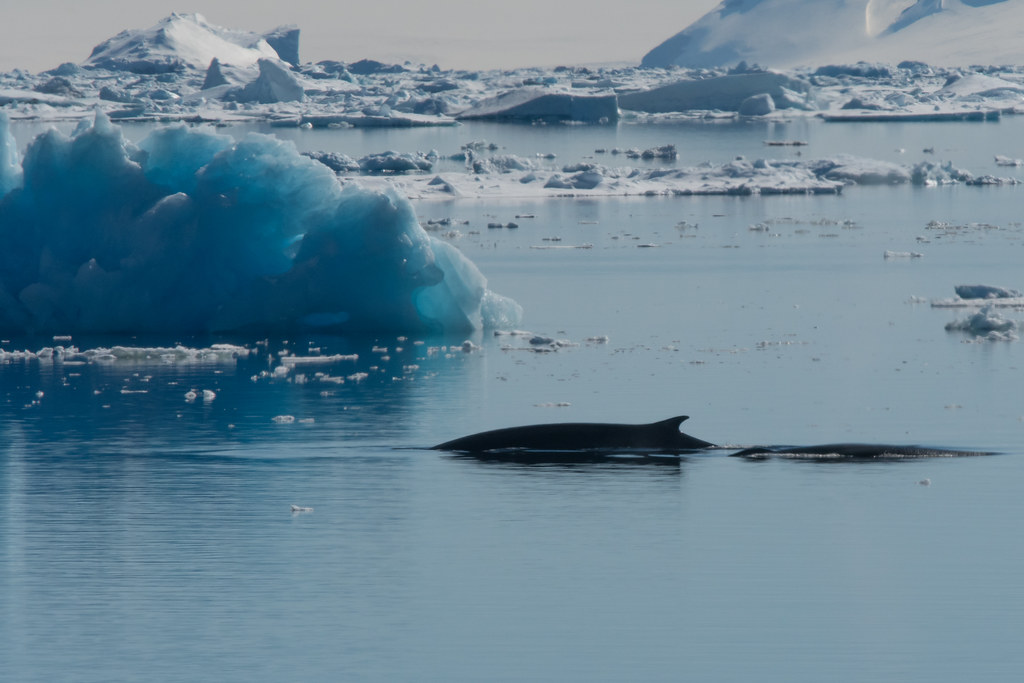This photograph, likely taken in the Antarctic, captures a serene, icy seascape on a sunny day. In the foreground, a dark, marine animal—possibly an orca or dolphin—emerges partially from the calm, reflective waters, with only about 10% of its body visible above the surface. To the left of the animal, a prominently blue iceberg appears recently flipped, revealing a deep aqua hue that resembles crystal. The background showcases snow-covered land and serene ice formations, contributing to the tranquil atmosphere. The high resolution and clarity of the image suggest it was taken with a professional camera, highlighting the stunning transparency and colors of the surrounding ice.